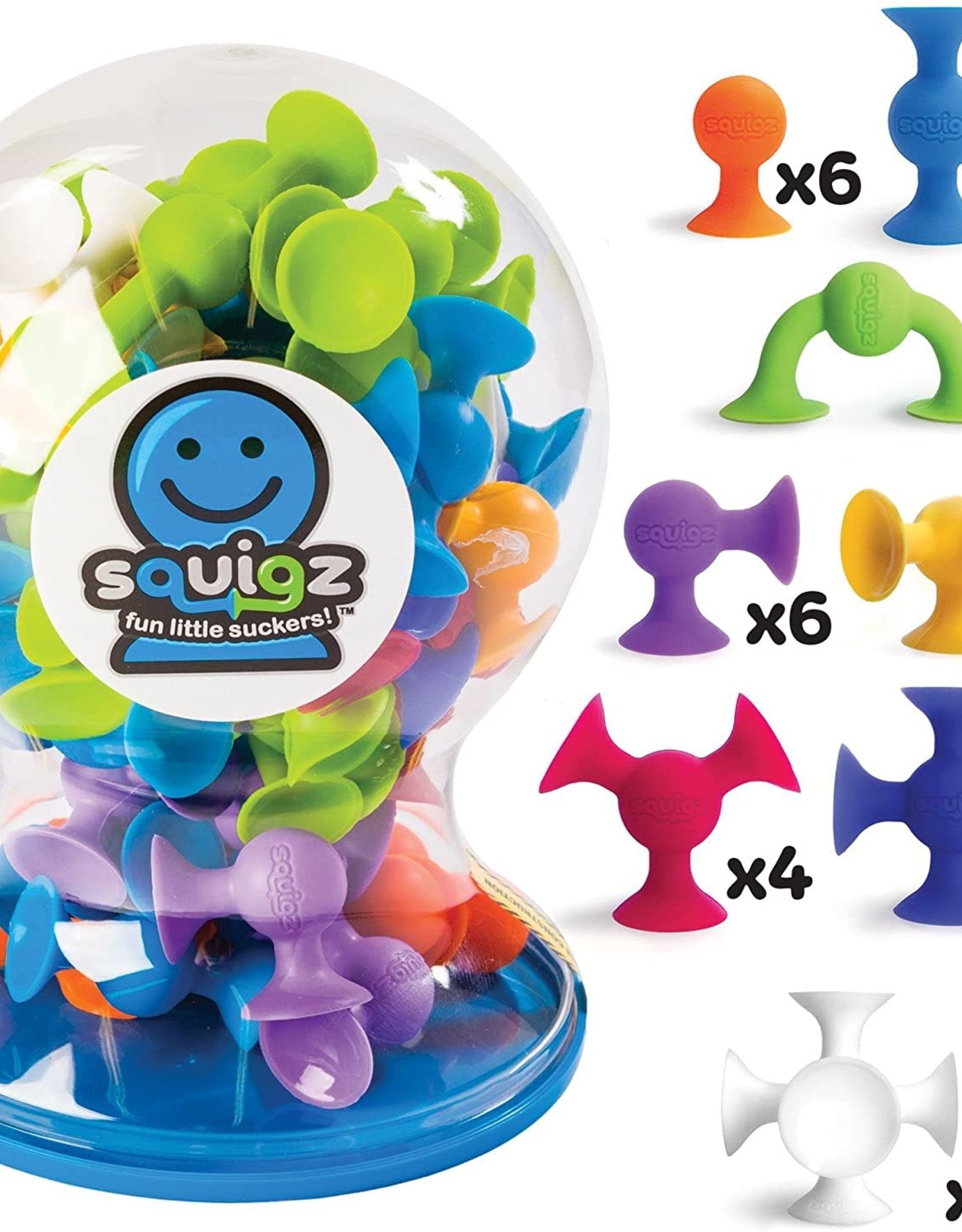The image is styled like a kid's toy advertisement and features a children's suction toy set called "Squigs Fun Little Suckers." The background is completely white, enhancing the clarity of the colorful elements. On the left-hand side, there is a clear plastic dome-shaped container with a blue base, filled with an assortment of vibrant toys in colors such as purple, green, pink, orange, and white. The container has a white circular label featuring a blue smiley face with a turquoise highlight, and the text "Squigs Fun Little Suckers." 

On the right-hand side, individual toys are displayed in a vertical column, showcasing various shapes and colors including orange, blue, green, purple, yellow, pink, and white. The numbers of each toy type are indicated with "X6" written between the top two and middle pairs, and "X4" between the lower pink and blue pair. Each toy has small, suction cup-like attachments labeled "Squigs," which are depicted in detailed views to highlight their design and functionality. This visually appealing layout shows both the sealed packaging and the individual components, making it clear for potential buyers what they are getting.